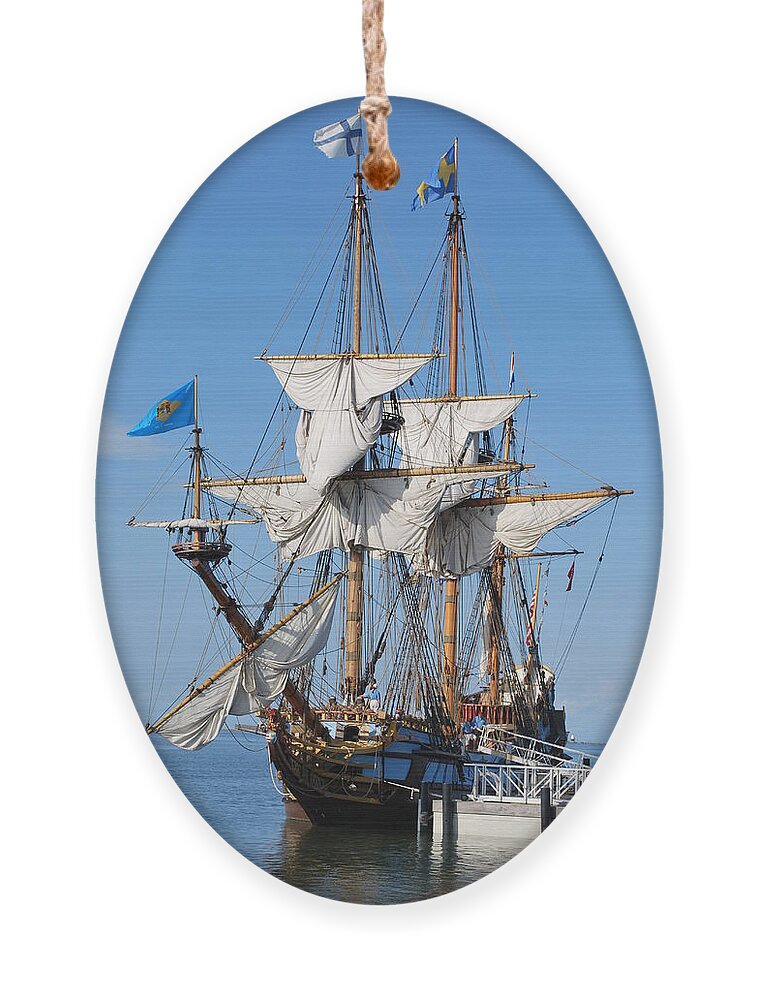The image is shaped like an oblong mirror or ornament, suspended by a rope through a hole at the top. It features a vividly bright blue sky covering three-fourths of the composition, with the bottom fourth depicting water. Dominating this aquatic scene is a large, white, and gold-trimmed pirate-like ship. The ship, anchored beside a barely visible wooden dock, boasts six distinctly white sails currently hoisted, three of which are mounted on three central masts. Affixed to these masts are multiple flags—the most prominent being a light blue flag with a gold crest, presumably inscribed with the letters "RH". There are two additional flags at the top, one showing a blue cross on a white background, and another, more indistinct, blue and yellow flag fluttering in the wind. The entire composition, possibly evoking a historical era ranging from the 7th to 18th century, is teeming with intricate ship rigging and a ladder ascending one side of the vessel, enhancing its detailed maritime aesthetic.